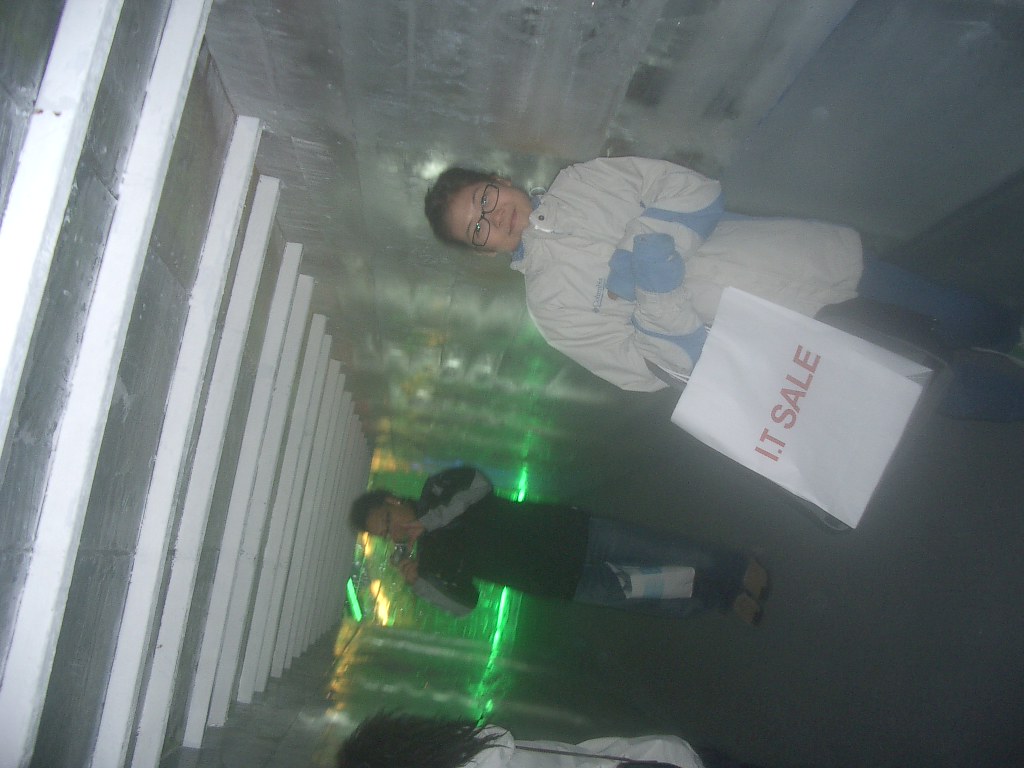This detailed photograph captures three Chinese individuals indoors, each immersing in an apparent shopping spree. At the forefront, a woman wearing a white coat with light blue sleeves and blue pants stands with a shopping bag that declares "IT Sale." The bag, a white paper version with handles, is looped around her arm as she strikes a pose that suggests she might be feeling a bit chilly. Her hands are gloved, and she sports black-framed glasses with clear lenses, complementing her black hair.

Behind her, a man is engrossed in his phone, holding it up with both hands, necessitating him to squeeze his shopping bag between his legs. He wears a black jacket with gray stripes on the sleeves, blue jeans, and brown boots, with his appearance highlighted by glasses that match the woman's in frame and lens clarity. His ensemble is completed with earrings, adding a touch of personal flair.

Not far from him, another woman can be seen wearing a white jacket, her dark hair harmonizing with light blue-colored sleeves, and blue pants, similar to the first lady's outfit. This photograph is taken at a peculiar angle, necessitating a 180-degree rotation for a straightforward view. Additionally, a green light emanates from the background, casting an unusual hue over the scene.